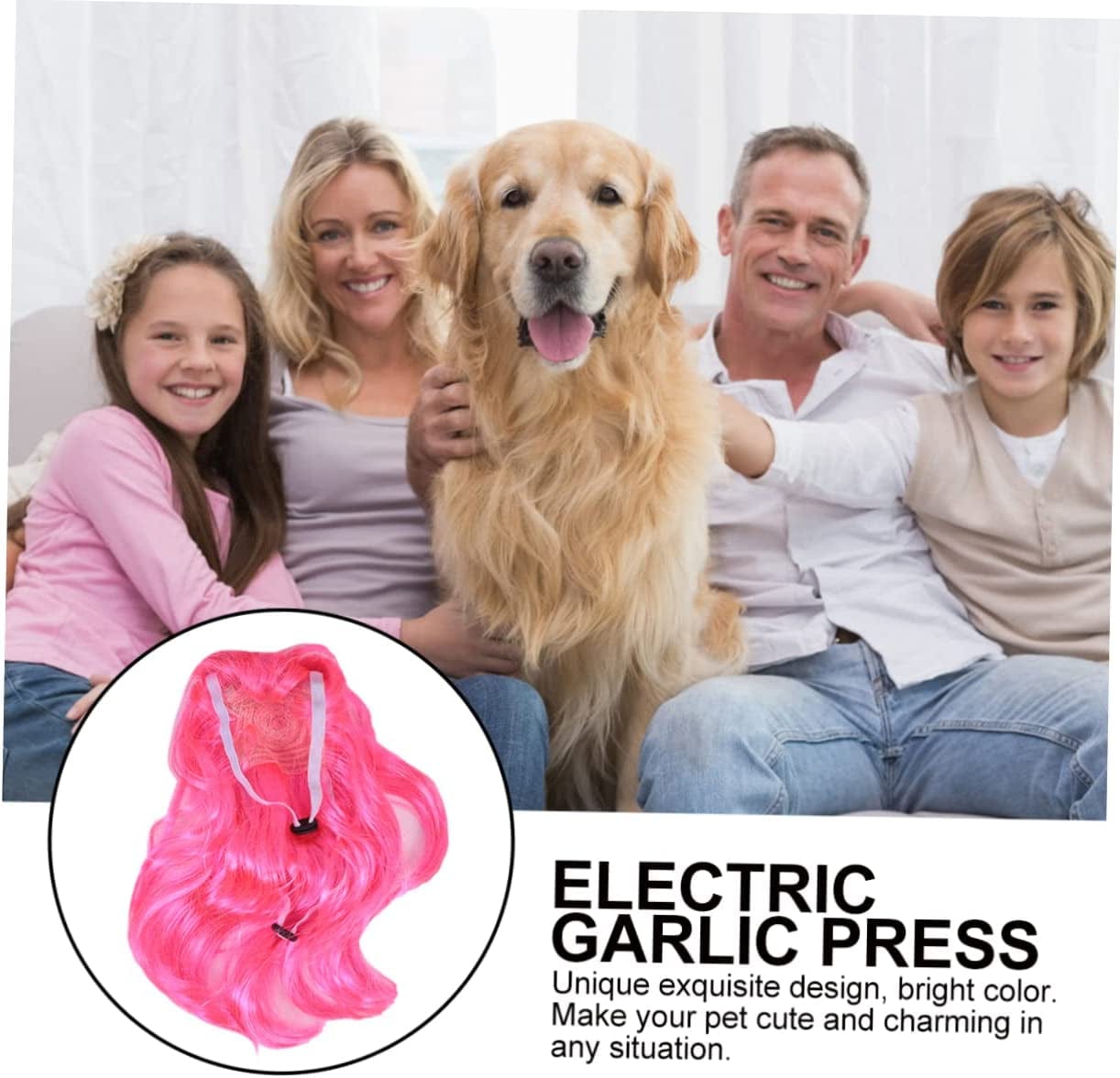In this color photograph, a jubilant family sits together on a sofa adorned with white curtains in the background. On the left, a young girl with long brown hair wears a pink long-sleeved top and jeans, her smile accentuated by a flowered headband. Beside her sits a woman with shoulder-length blonde hair in a gray shirt, her hand affectionately placed on a blissful golden retriever in the center. The dog, mouth open in apparent joy, bridges the space to a man with short hair and no beard, dressed in a white button-up shirt and light denim jeans. On the far right, a child with short blonde hair and a brown Henley shirt gazes pleasantly at the camera. All family members direct their smiles toward the lens, exuding warmth and togetherness. At the bottom left corner of the image is an inset of a pink wig, alongside the text "ELECTRIC GARLIC PRESS. Unique, exquisite design, bright color. Make your pet cute and charming in any situation."